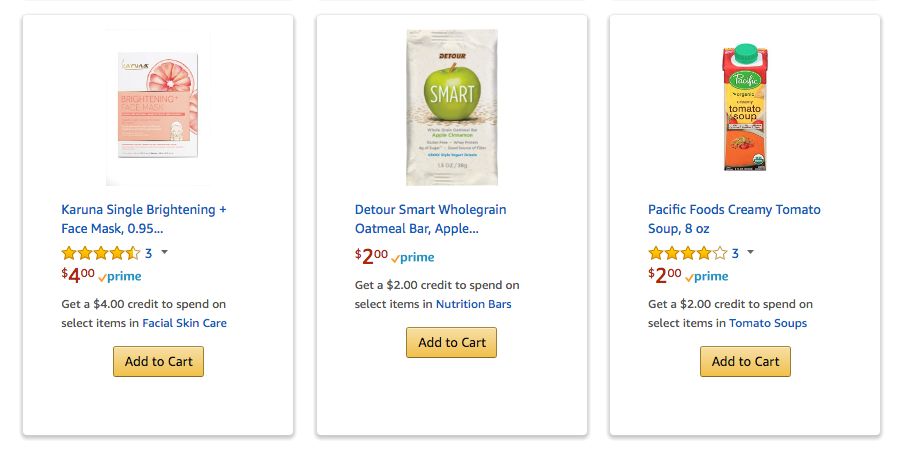Below is a detailed and clean caption for the given description:

---

**Screenshot of Amazon Product Listings:**

The image depicts a screenshot from Amazon displaying three different product offerings, each available for purchase with specific deals attached. 

1. **Karuna Single Brightening Face Mask (0.95 oz):**
   - **Price:** $4 on Prime
   - **Product Description:** Comes in a box featuring a design with a pink lemon.
   - **Customer Reviews:** Three reviews with an average rating of 4.5 stars.
   - **Deal:** Receive a $4 credit to spend on select facial skincare items.
   - **Option:** Add to Cart

2. **Detour Smart Whole Grain Oatmeal Bar, Apple:**
   - **Price:** $2 on Prime
   - **Product Description:** Packaged in a box adorned with an apple illustration.
   - **Deal:** Receive a $2 credit to spend on select nutritional bars.
   - **Option:** Add to Cart

3. **Pacific Foods Creamy Tomato Soup (8 oz):**
   - **Price:** $2 on Prime
   - **Product Description:** Comes in a red carton with a green top.
   - **Customer Reviews:** Three reviews with an average rating of 4 stars.
   - **Deal:** Receive a $2 credit to spend on select tomato soup items.
   - **Option:** Add to Cart 

Each product features a promotional offer where customers can earn credits towards future purchases in their respective categories, enhancing the value of these deals.

---